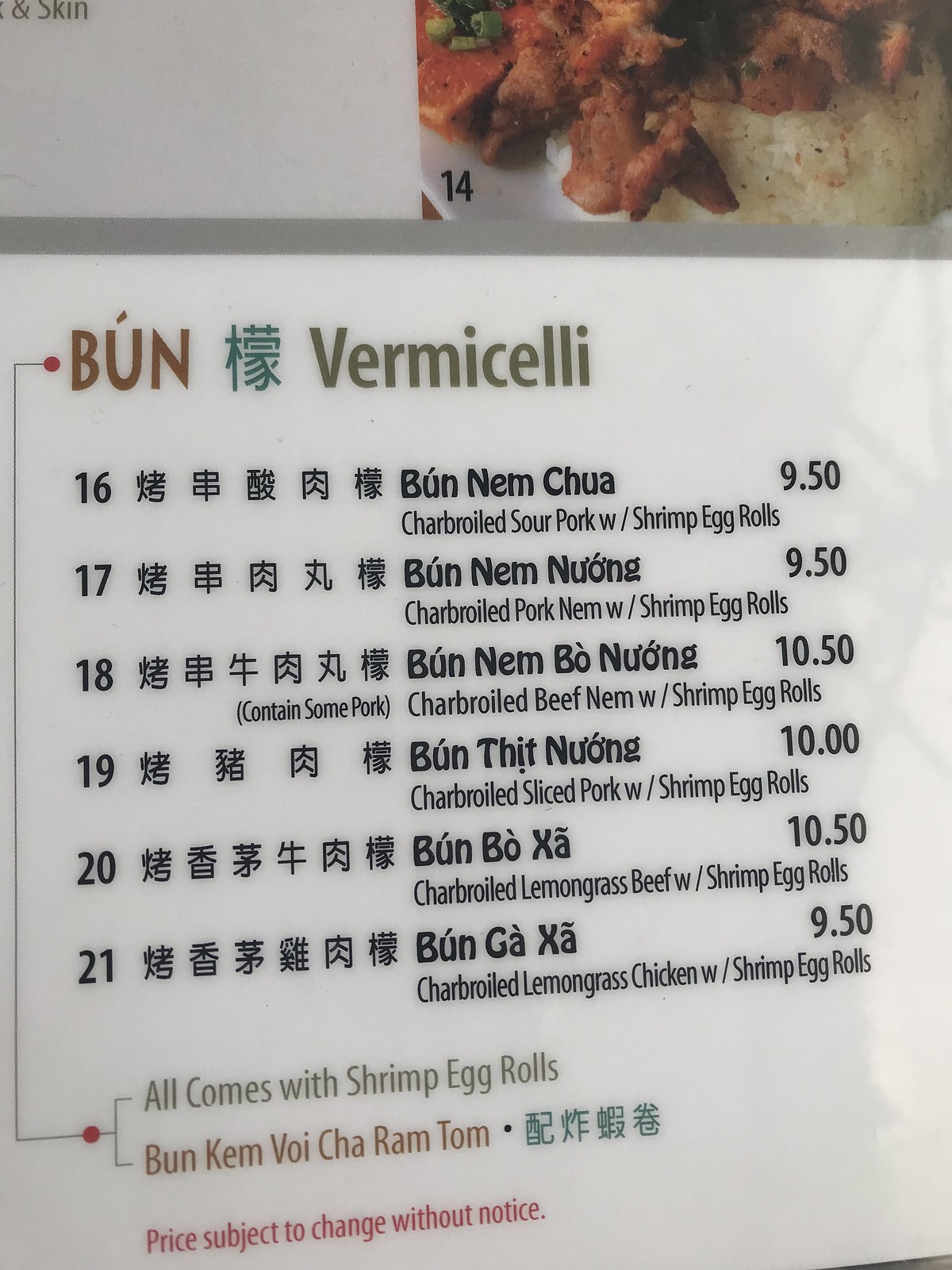This image captures a section of a laminated, white Vietnamese menu titled "Bun [Asian Character] Vermicelli." In the upper right corner of the image, a photo of a dish labeled "14" showcases fried brown pieces of meat, likely chicken, served on a bed of white rice mixed with cut vegetables. Though the number 14 refers to another sheet, the visible part of the menu starts at number 16 and continues to number 21. Each item includes the dish number, Asian characters, the English name, and a brief description. For instance, number 16, "Bun Nem Chua," is described as charbroiled sour pork with shrimp egg rolls. Prices for each item are listed to the right.